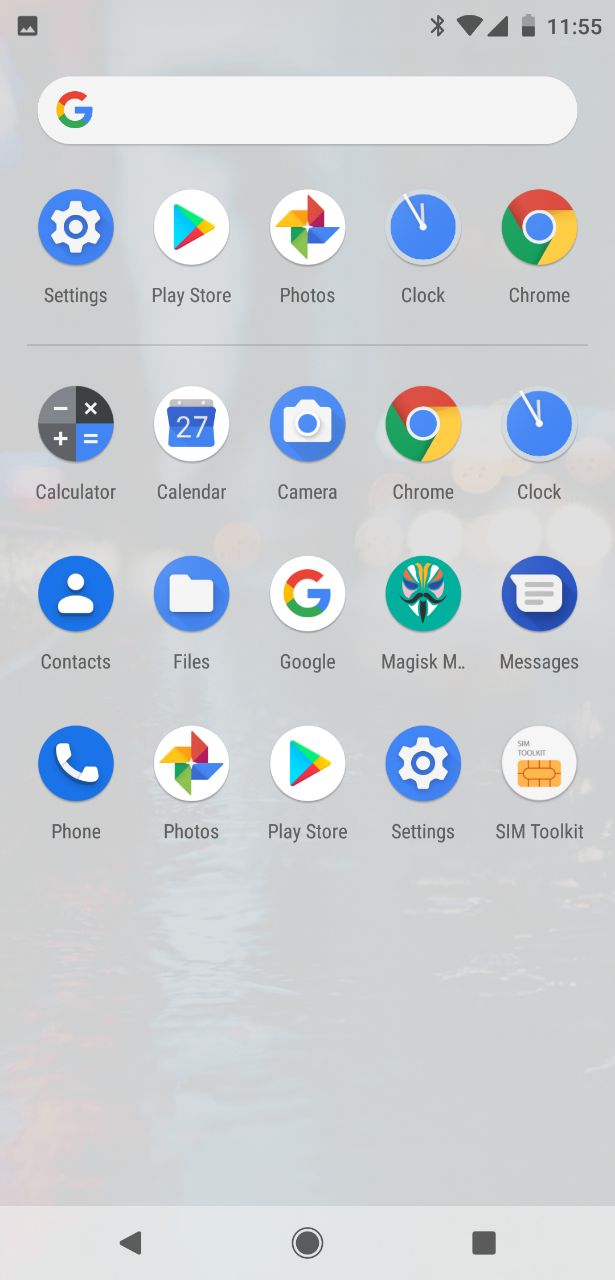This is a detailed screenshot showcasing a variety of Google apps and other applications. At the top of the image is the iconic Google search bar, easily recognizable by the multicolored (red, yellow, green, and blue) 'G' logo within a white search bar. 

Moving to the first row of app icons, we have:
1. **Settings**: Depicted by a blue circle featuring a white gear icon.
2. **Play Store**: Represented by the traditional multicolored triangle logo.
3. **Photos**: Illustrated with the Google Photos multicolored pinwheel icon.
4. **Clock**: Shown with an image of a clock face.
5. **Chrome**: Identified by the well-known round Chrome browser icon.

In the second row of app icons, the arrangement includes:
1. **Calculator**: Displays the classic calculator icon featuring mathematical symbols such as minus, multiplication, plus, and equal sign.
2. **Calendar**: Shows the date '27' on its icon.
3. **Camera**: Illustrated with a camera icon.
4. **Chrome**: Repeated again with the same Chrome browser icon.
5. **Clock**: Appears a second time with the same clock face icon.

On the third row of app icons, we find:
1. **Contacts**: Depicted by a blue circle with a white silhouette of a person.
2. **Files**: Represented by another blue circle, this time featuring a white folder icon.
3. **Google**: Shown with the iconic multicolored 'G' logo.
4. **Magisk**: Displayed with a teal circle containing a white mask with a mustache and goatee.
5. **Messages**: Identified with an icon representative of messaging apps.

Finally, the bottom row of app icons consists of:
1. **Phone**: Illustrated by a blue circle with a white phone receiver icon.
2. **Photos**: Reappears with the Google Photos pinwheel icon.
3. **Play Store**: Again shown with the multicolored triangle.
4. **Settings**: Repeated with the blue circle and white gear.
5. **SIM Toolkit**: Included as the final application in this row, typically represented by an icon pertinent to carrier settings and SIM management.

This comprehensive lineup of apps is neatly arranged in a four-row grid format against a backdrop typical of a smartphone home screen.